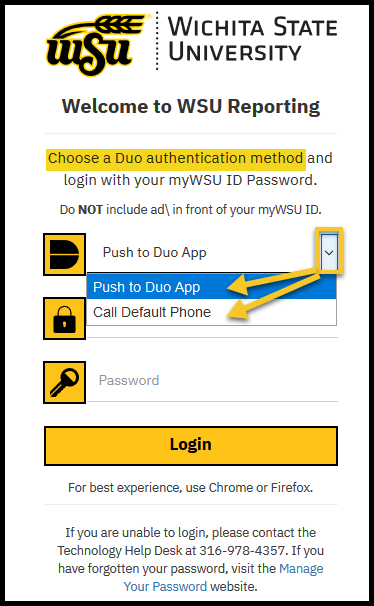The image features a white box with a black border. At the top, there is a black text "WSU" with a gold border surrounding each letter. Emerging from the "W" is a graphic of a wheat stalk. To the right of this, "Wichita State University" is written in black text.

Below this, the text "Welcome to WSU Reporting" is displayed. Further down, the instructions read, "Choose a Duo authentication method and log in with your MyWSUID password." Another instruction below this warns in all caps, "DO NOT include 'add/' in front of your MyWSUID."

Further instructions show a yellow arrow pointing towards the instruction "Push the Duo App," and another yellow arrow directs attention to "Call default phone."

At the bottom of the box, there is a yellow rectangle with a black key icon inside it. Beside this, a box labeled "Password" is displayed. Beneath these elements lies another yellow rectangle with a black border and the word "Login" in black text centered in the middle.